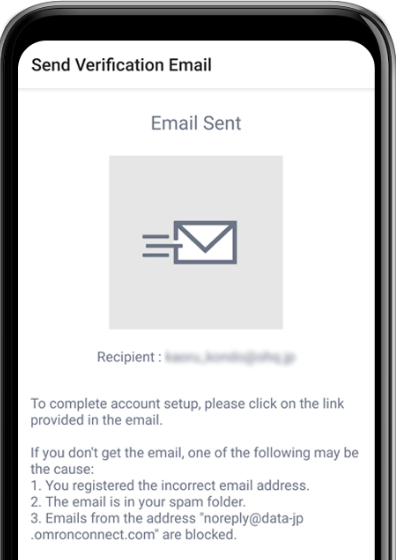This digital image features a partially visible cell phone with a black and silver border. The bottom left, bottom right, and bottom center of the cell phone are cut off, obscuring the complete view of the device and any additional content. The focus of the image is a screenshot displayed on the cell phone screen.

In the top left corner of the screenshot, in bold black text, it reads "Send Verification Email." Below this header is a gray horizontal line. Beneath the line, in gray text against a white background, it states "Email Sent," which can be challenging to read due to the contrasting colors.

Centered in the image, there is a gray box containing an icon of a sent email, depicted as an envelope with three movement lines to the left, indicating motion. Below the icon, the text "Recipient:" is displayed, but the actual recipient's name has been intentionally erased by the user who captured the screenshot.

Further down, the text instructs, "To complete account setup, please click on the link provided in the email. If you don't get the email, one of the following may be the cause:" followed by three potential reasons:
  1. You registered the incorrect email address.
  2. The email is in your spam folder.
  3. Emails from the address noreply@data.jp.omronconnect.com are blocked.

The emphasis is both on the process of sending a verification email and troubleshooting steps if the email is not received.